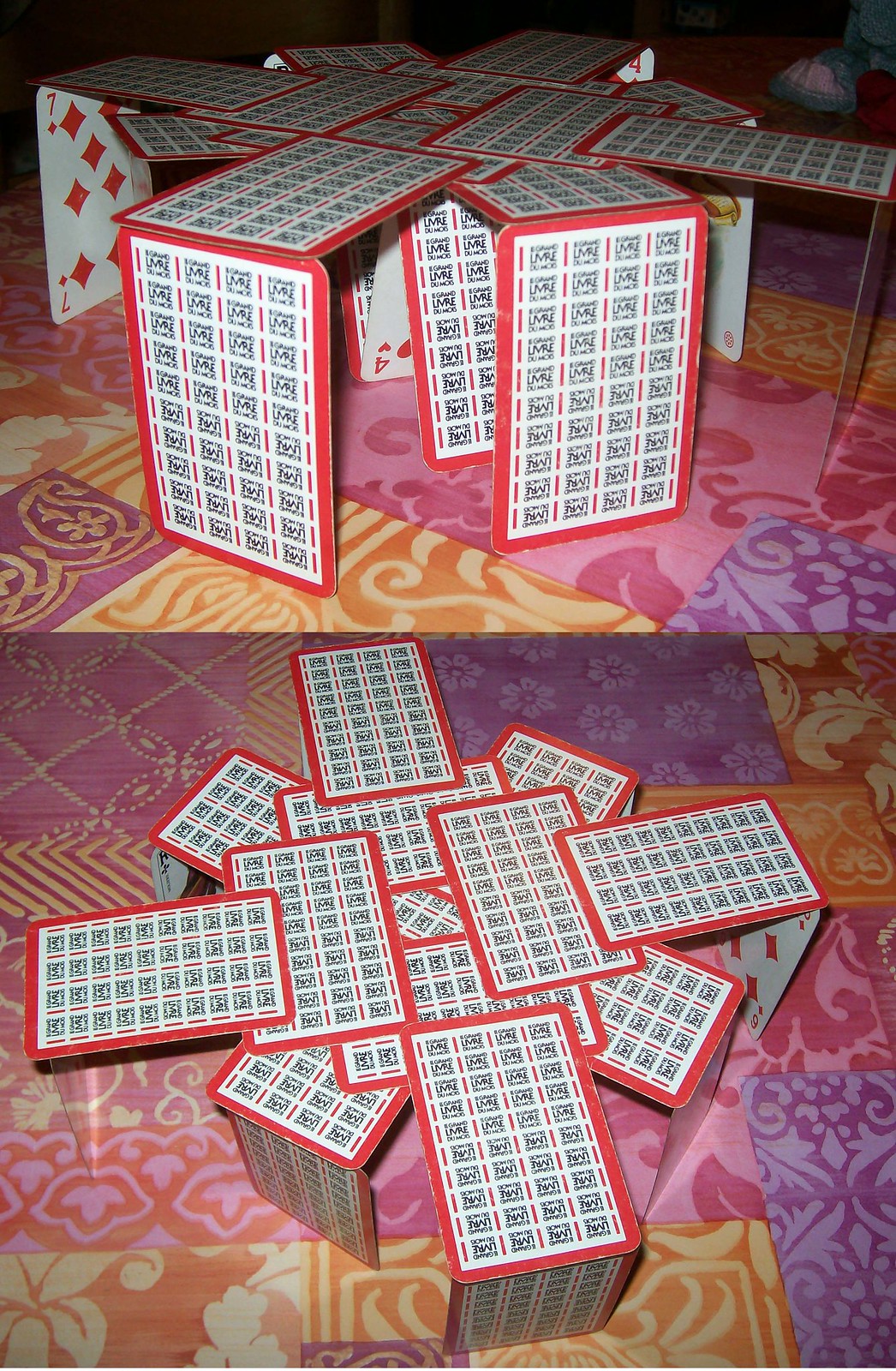Here’s a detailed and cleaned-up descriptive caption for the image:

---

The image consists of two photographs, one positioned above the other, both showcasing a unique house of cards. In the top photograph, the house of cards is built to one level, with six cards forming the structure. These cards are positioned upright, facing the viewer, and a pair of cards is laid flat on top, acting as the roof. The arrangement spreads outward from a central point, creating a hexagonal pattern.

The structure rests on a vividly colorful surface, possibly a tablecloth or carpet, adorned with blue, pink, yellow, and purple designs that resemble a floral pattern. 

The bottom photograph presents the same house of cards from a top-down perspective, offering a detailed view of the arrangement. The cards themselves are quite unusual — the backs are decorated with rows of black designs set between red lines, which might be mistaken for QR codes at a glance. Behind the house of cards, a seven of diamonds from a regular playing card deck is visible, adding to the intrigue of the setup.

---

This revised caption provides a comprehensive description of both photographs and their contents.